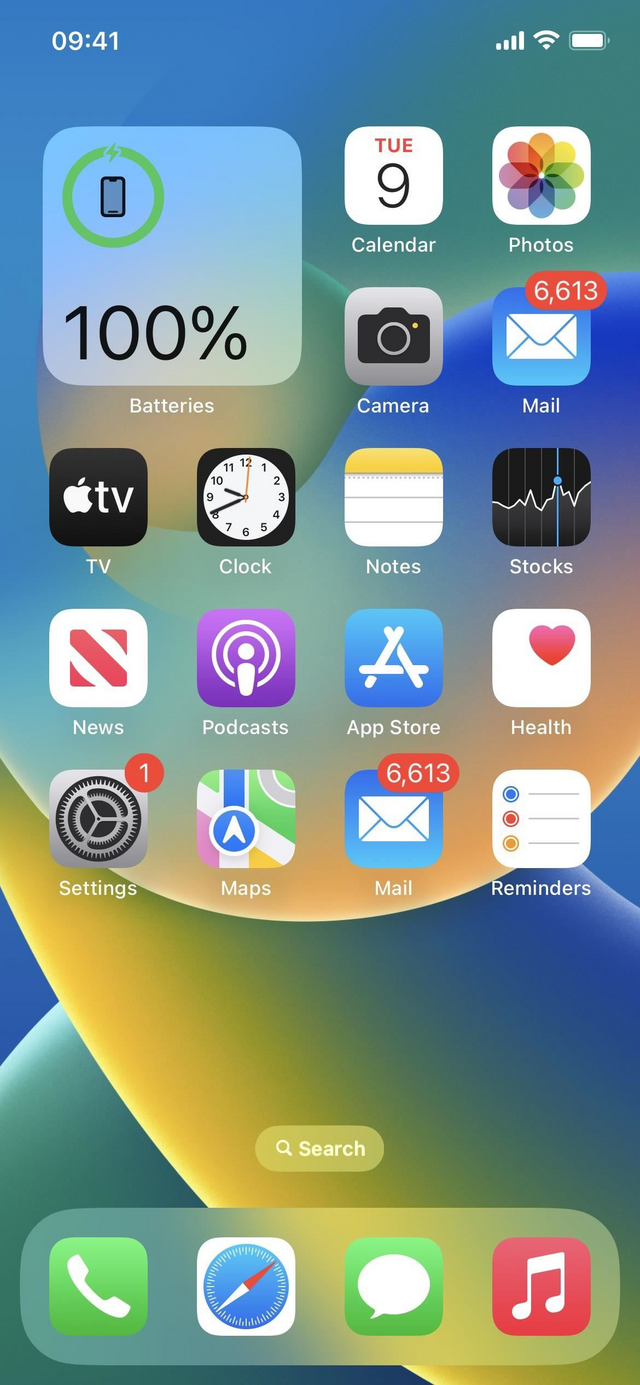This image depicts the home screen of someone's smartphone. The background transitions through a blend of colors, beginning with blue in the upper left corner, shifting to green in the middle, merging into blue and yellow, transitioning again into yellow and blue, and finally settling into a greenish-blue hue at the bottom left.

In the top-left corner, the time is displayed as 9:41, accompanied by a battery icon indicating a full charge at 100%. A phone icon with a green circle is also visible, reinforcing the full battery status.

The home screen showcases a variety of apps arranged neatly. At the top, the Calendar app displays the date as Tuesday the 9th, followed by icons for Photos, Camera, and Mail, which reveals an overwhelming 6,613 unread emails. Additional apps include Apple TV, Clock, Notes, Stocks, News, Podcasts, App Store, Health, Settings (highlighted with a notification indicating one unchecked item), Maps, Mail, and Reminders.

At the bottom of the screen, there is a dock containing the user's frequently used apps: Phone, Safari, Text Messaging, and Music. Just above this dock, a small search bar is conveniently placed, providing easy access for quick searches.